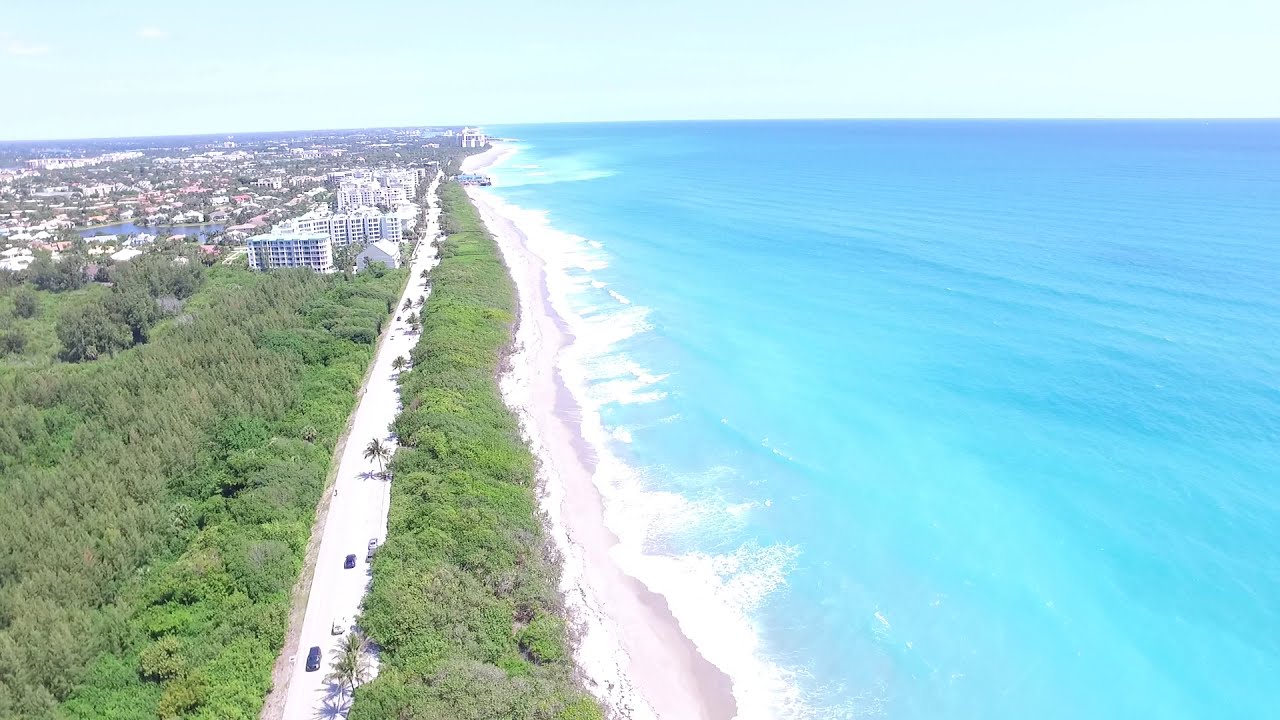This image is an aerial view of a strikingly beautiful tropical coastline. On the right half of the picture, the endless expanse of the ocean is a mesmerizing clear aquamarine blue, resembling a perfectly serene swimming pool. The waves gently crash against the white sandy beach that stretches alongside the coast, with the blue sky above seamlessly merging with the water in the distance. 

In the background, on the left-hand side of the picture, stands a bustling cityscape filled with large hotels, condos, and houses. A long, straight four-lane road runs down the center of the image, separating the lush greenery of trees and brush from the coastline. Along the road, towards the left, the landscape is dotted with a vast array of green trees and vegetation, creating a vivid contrast against the urban backdrop.

To the right of this road, a swath of dense foliage provides a natural barrier between the city and the pristine beach. Between the buildings and the road, there's a noticeable pond, likely fed by the ocean. The top of the picture captures a clear blue sky, enhancing the tropical ambiance of this scenic coastline. This detailed view encapsulates the tranquility of the ocean, the serene greenery, and the vibrant energy of the city, harmoniously coexisting in one picturesque setting.